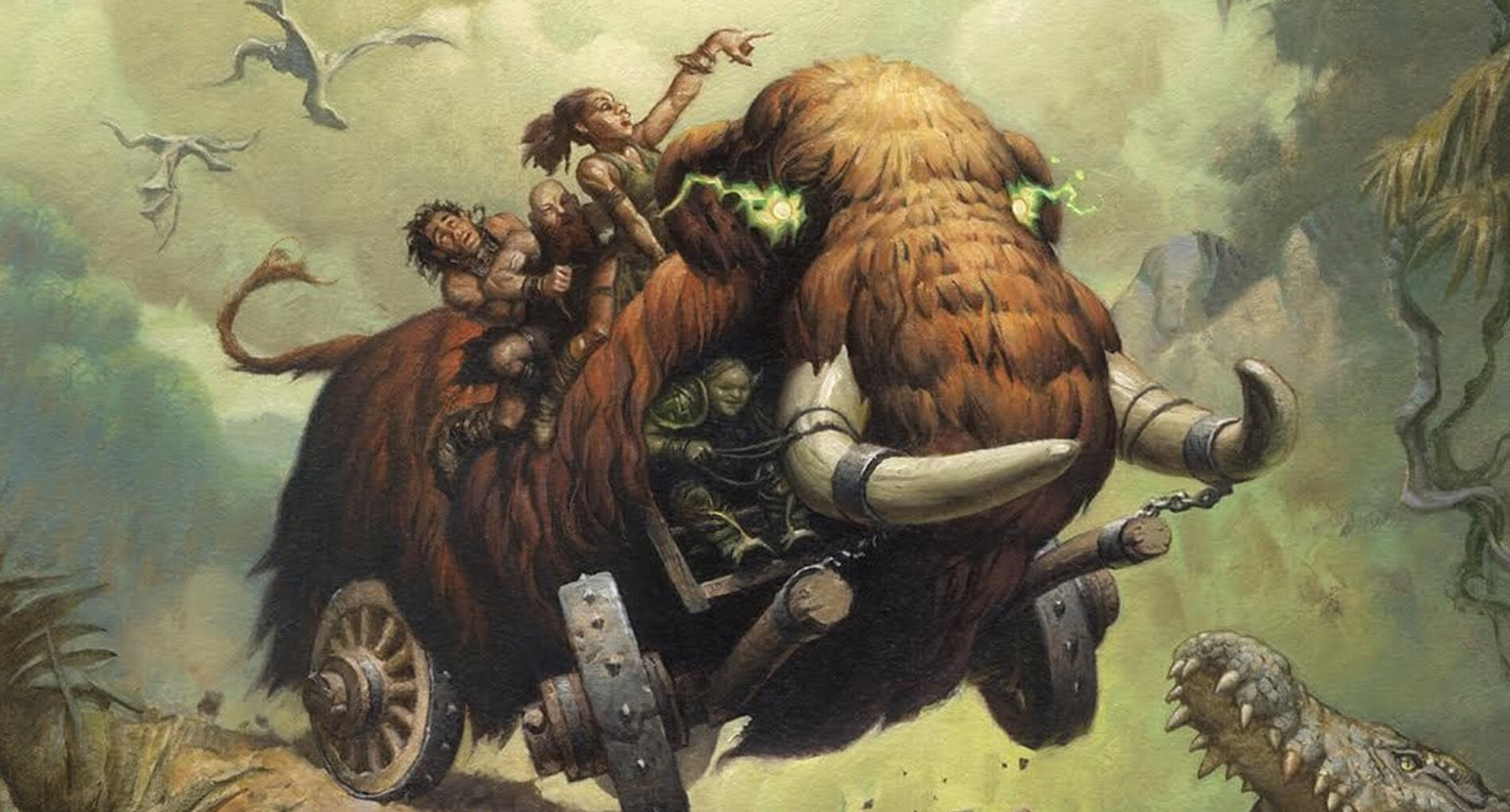In this animated, fantastical painting, a futuristic vehicle, crafted to resemble a woolly mammoth, features prominently. The mammoth-like creature, covered in brown fur, has enormous silver tusks and striking yellow eyes that emit sparks, giving it an electrified appearance. Notably, its feet are replaced with metal wheels, emphasizing its mechanical nature. A troll-like figure, embedded near its tusk, appears to be steering the mammoth, while atop its back sit three passengers: a spirited young girl pointing to the right with her mouth open, a middle-aged balding man, and a terrified man clinging on with black hair. Above them, the sky is filled with silver flying creatures, resembling pterodactyls, amidst a backdrop of yellow to dark green clouds. Vines creep down the painting's right side, hinting at a lush, forested environment below. A massive crocodile or alligator with its jaw agape lies beneath the mammoth's leap, adding a sense of imminent danger and dynamic motion to the scene.